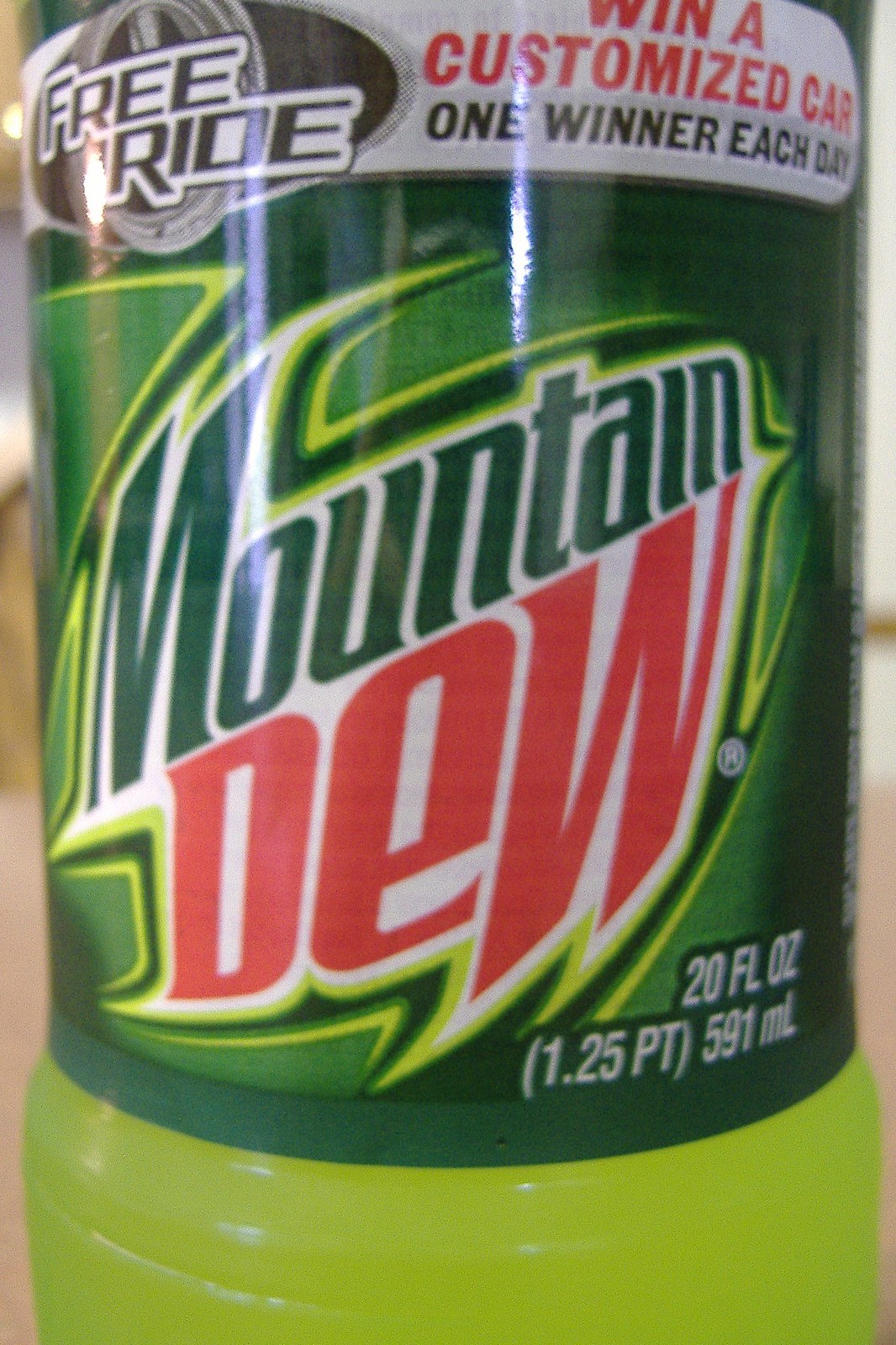This is a close-up portrait mode photograph of a 20-ounce bottle of Mountain Dew, showcasing the label in vivid detail. The bright lime-green liquid of the soda is visible through the transparent plastic at the bottom of the bottle, emphasizing its vibrant color. The label itself dominates the image with a greenish background accented by lightning bolt-like borders around the large Mountain Dew logo centrally positioned. Above the logo, a promotional advertisement is displayed prominently in white with red and black text. The ad consists of two parts: on the left, "Free Ride" is written over an image of a hubcap, and on the right, "Win a customized car" is featured in red text with "One winner each day" in black text beneath it. Additionally, the bottom right corner of the label details the bottle's contents as "20 fluid ounces" (equivalent to "1.25 pt" or "591 milliliters").